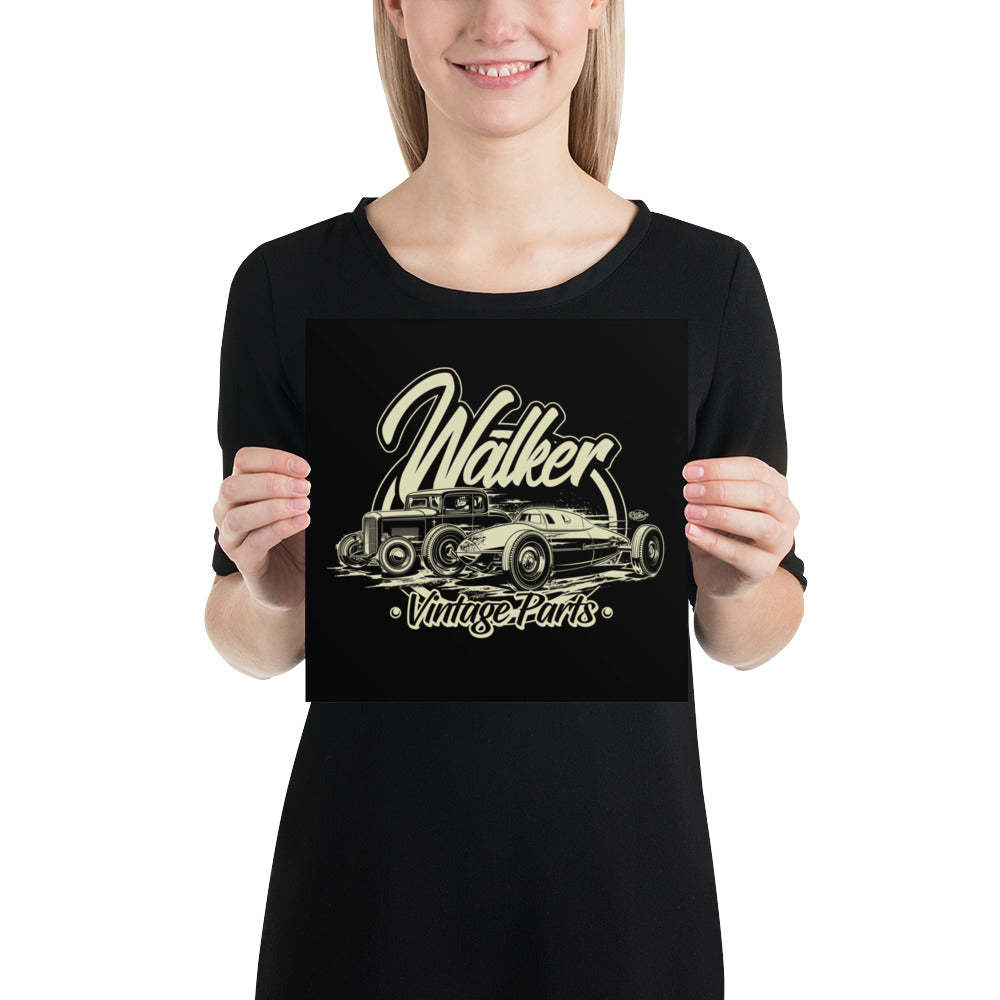This color photograph is in portrait orientation and features a young woman depicted from just below her eyes to her mid-hip. She has straight blonde hair, which is pushed behind her ears, and she is sporting pink lips. She wears a simple black dress with a wide neck and half sleeves that extend to her elbows. The subject holds a black square in front of her chest. The square displays a graphic in cream-colored cursive letters that reads "Walker Vintage Parts," with "Vintage Parts" written beneath "Walker." Between the words is a circle containing an illustration of two vintage cars from the 1940s, positioned as if traveling in opposite directions. The woman's facial expression is inviting, and the overall style of the image is photographic representational realism, highlighting the proposed design on the black square she is holding.